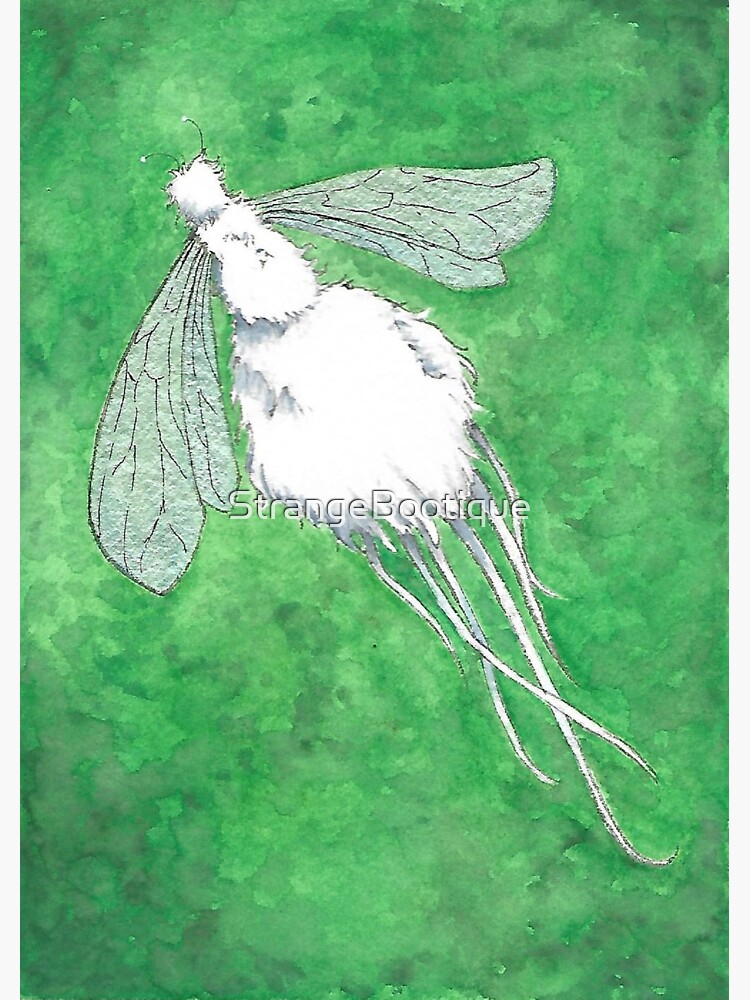This detailed drawing, presented in a portrait layout with a green, mottled background varying from darker greens in the corners to different shades of lighter green and cream in the center, features a unique insect-like creature prominently positioned diagonally from the upper left to the lower right. Viewed from an overhead perspective, the creature's body is segmented into three parts – a smaller head, a medium-sized torso, and a larger rear end. The wings, thin with delicate leaf-like patterns and bordered in black, are semi-translucent with the background shining through slightly. The creature sports black and white-tipped antennas and has six substantial appendages trailing from its rear, resembling spider threads or legs. The entire image exudes an artistic and whimsical feel, further accentuated by the text "Strange Boutique" inscribed in white across the center.